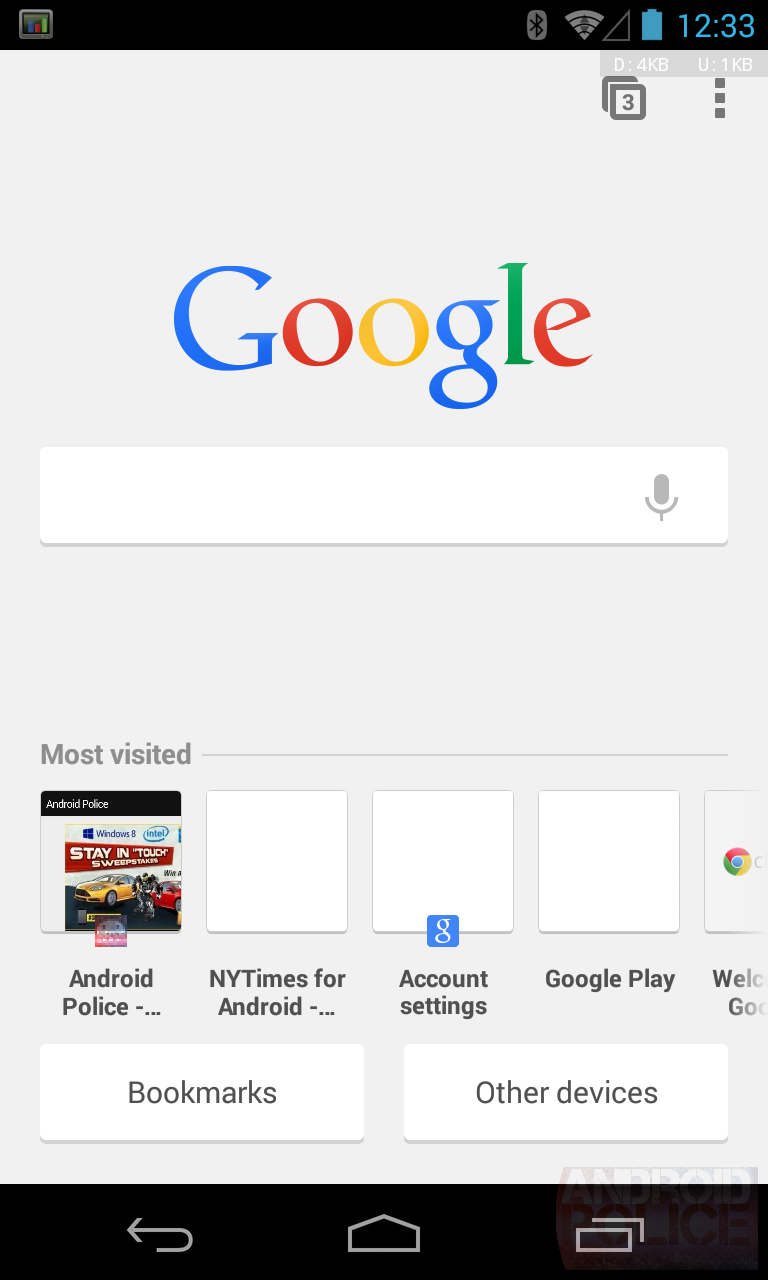This image is a screenshot of a Google search homepage. At the center of the screen is the iconic Google logo, featuring the word "Google" spelled in various colors: a blue capital 'G', red 'o', yellow 'o', green 'l', and a red 'e'. Below the logo is a search bar where users can input their search terms. Underneath the search bar is a section titled "Most visited," displaying a series of thumbnails.

The first thumbnail shows an image with two sports cars, one red and one yellow, with the title "stay in the know." Below this image, the text reads "Android Police." Next to this thumbnail are others labeled, but without images, such as "New York Times for Android."

Another thumbnail labeled "Google Account Settings" features a small blue square with a white 'G' inside, partially overlapping the bottom edge of the first thumbnail. There is also a thumbnail for "Google Play." At the bottom of the screen are two tabs—"Bookmarks" and "Other devices"—facilitating further navigation.